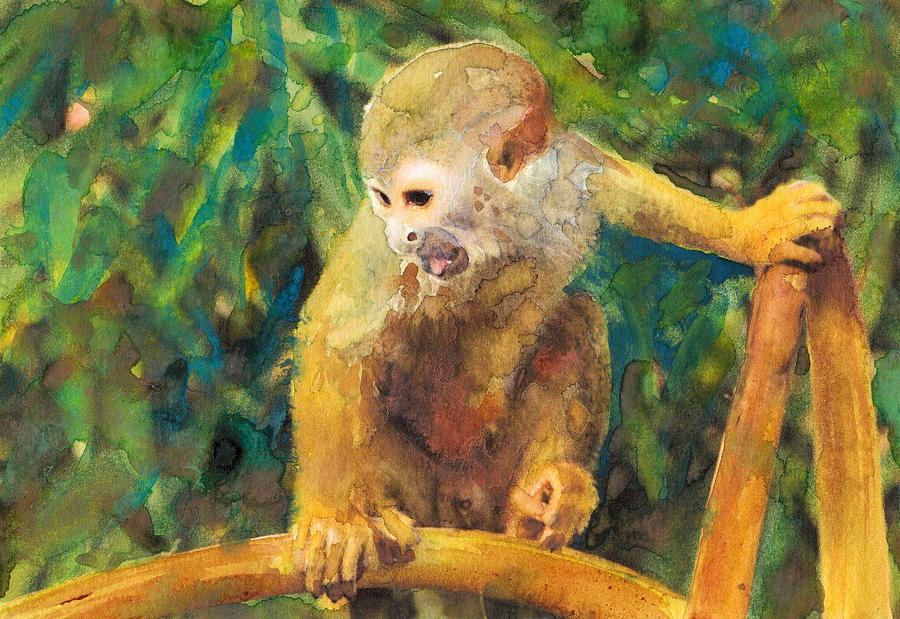The image appears to be a watercolor painting depicting a monkey, characterized by its abstract yet recognizable form. The monkey, featuring a palette of browns, yellows, creams, and rust-colored hues, is positioned in the center of the composition. Its face, turned to the side, shows black eyes, brown lips, and a little pink tongue sticking out, suggesting it might be making a noise. It has a white face and brown ears, with subtle hints of green in its overall coloration. The monkey is holding onto a tree branch with its feet, and one hand grips another vertically oriented branch, forming an upside-down V shape toward the right of the image. The background is filled with a blend of greens, blues, yellows, and browns in random shapes, evoking the impression of leaves and foliage in the surrounding tree. The overall effect of the painting is somewhat abstract, giving it a splotchy and modeled appearance that conveys a sense of artistic interpretation rather than precise realism.